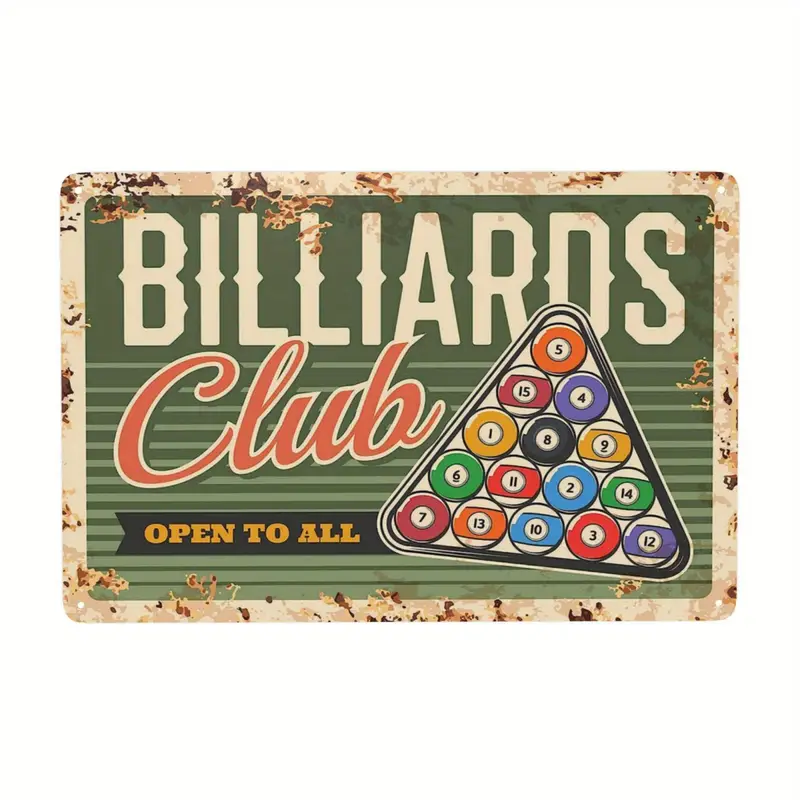The image depicts a horizontally aligned rectangular sign with four stylized rusted holes, suggesting an old bar sign. The outer border of the sign features a mixed pattern of light and dark brown spots resembling rust on a white background, with some spots intruding onto the central area of the sign. The main background is a solid sage green at the top, transitioning to lighter green with thin horizontal lines towards the bottom. 

In large, white, capitalized letters, the word "BILLIARDS" is prominently displayed at the top in an old Western-style font. Below it, the word "CLUB" appears in red cursive outlined in white, positioned towards the bottom left corner. Adjacent to this, in the lower left corner, a small black banner with gold (or orange) capital letters reads "OPEN TO ALL."

On the right side of the sign, a black-outlined triangle holds a set of pool balls arranged in a standard rack formation, featuring the specific numbers: 5, 15, 4, 1, 8, 9, 6, 11, 14, 7, 13, 10, 3, and 12. The detailed depiction of the balls and the text gives the sign a nostalgic, vintage appearance, with elements that may be digitally stylized to enhance its aged look.